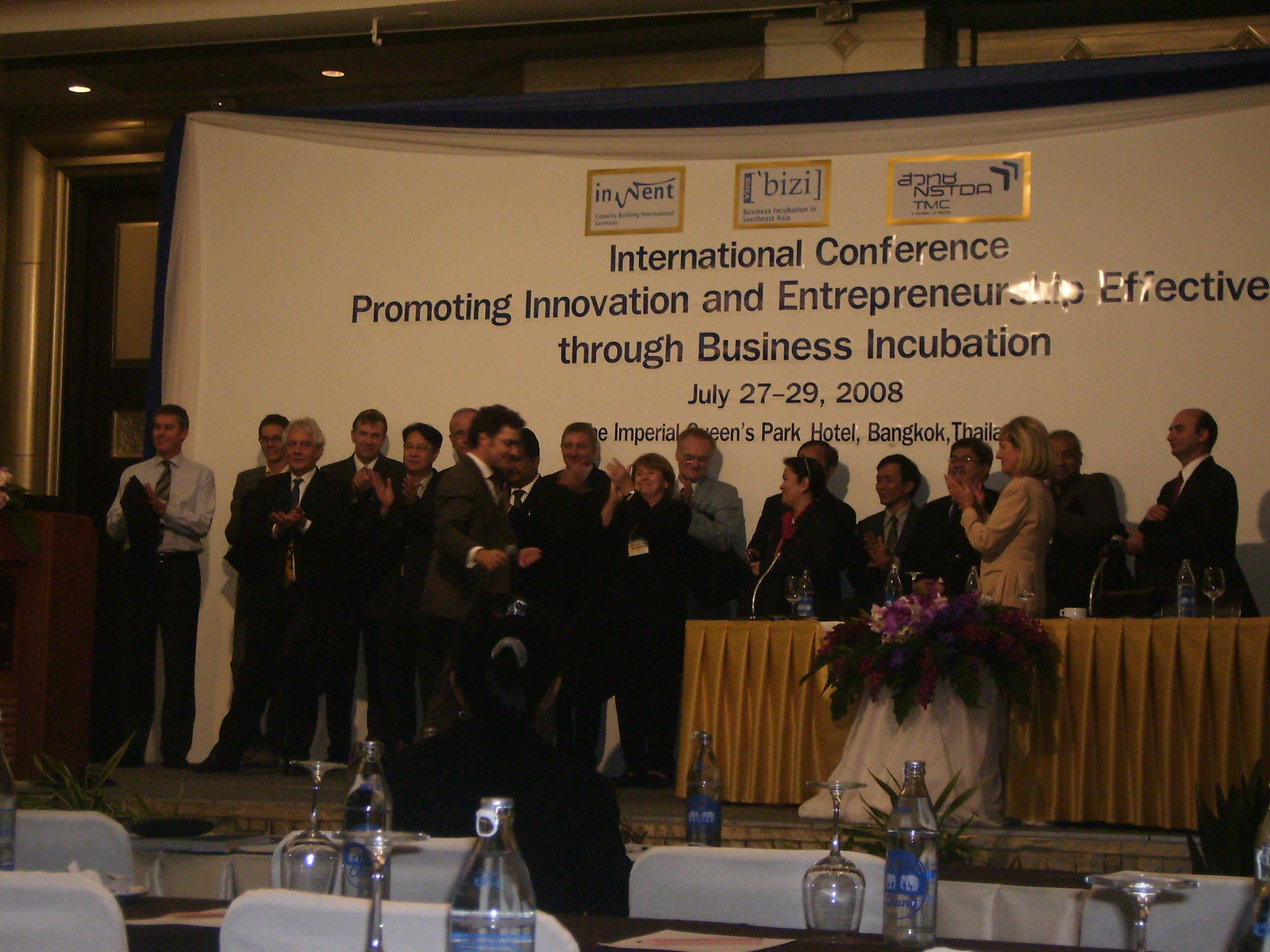The image captures an indoor setting at the Imperial Queens Park Hotel in Bangkok, Thailand, during the International Conference Promoting Innovation and Entrepreneurship held from July 27th to 29th, 2018. Dominating the frame is a large white banner behind a stage, which reads, "International Conference Promoting Innovation and Entrepreneurship, Effective through Business Incubation," with some parts partially obscured by lighting and a woman's hand. Below this main text are the dates and the venue details.

Center stage, a couple dozen people, many of whom are wearing name badges, stand lined up in front of the banner, with some applauding. They are dressed formally in suits and ties, capturing the professional atmosphere of the event. In the foreground, tables adorned with bottles of water, upside-down wine glasses, and additional glasses and microphones are visible, indicating that speeches were likely given before the group gathered for a photograph. The setup implies a formal conference environment, highlighted by other people walking towards the stage. The overall colors seen in the photo include gold, white, lavender, black, beige, gray, and blue.